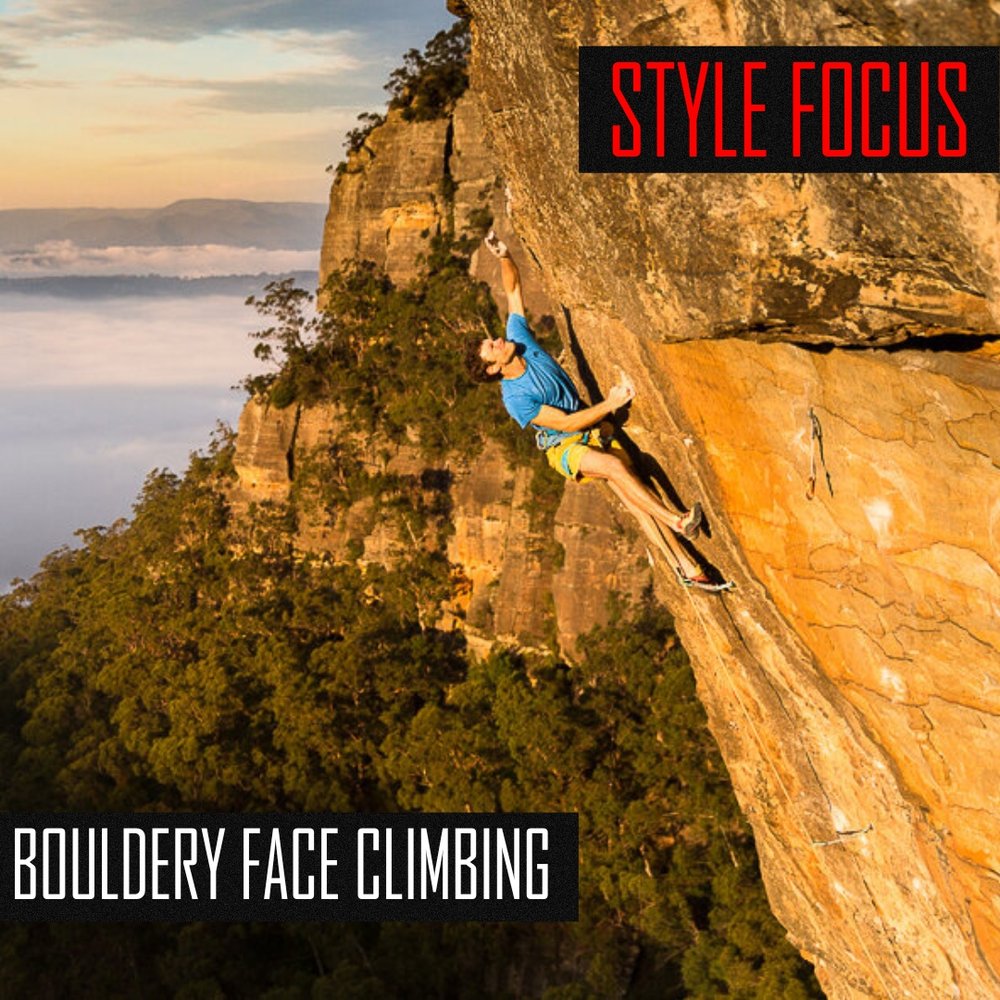The image appears to be a magazine cover featuring a striking photograph of a man engaged in rock climbing up a sheer, orange-tinged rock face, likely taken in the early morning due to the distinctive shadows and light. The climber, a slim man with short, dark hair, is sporting a blue shirt and bright yellow shorts, with what looks like white chalk on his hands. Notably, he doesn't seem to be using any visible safety equipment or cables. The natural setting in the background is composed of a serene body of water and a scattering of trees. The magazine cover includes text; "Style Focus" is prominently displayed in red capital letters within a black box at the top right, and the phrase "Bouldery Face Climbing" is placed in white letters on a black background at the bottom left. The overall palette of the image features a combination of brown, green, red, black, blue, yellow, orange, and white colors.